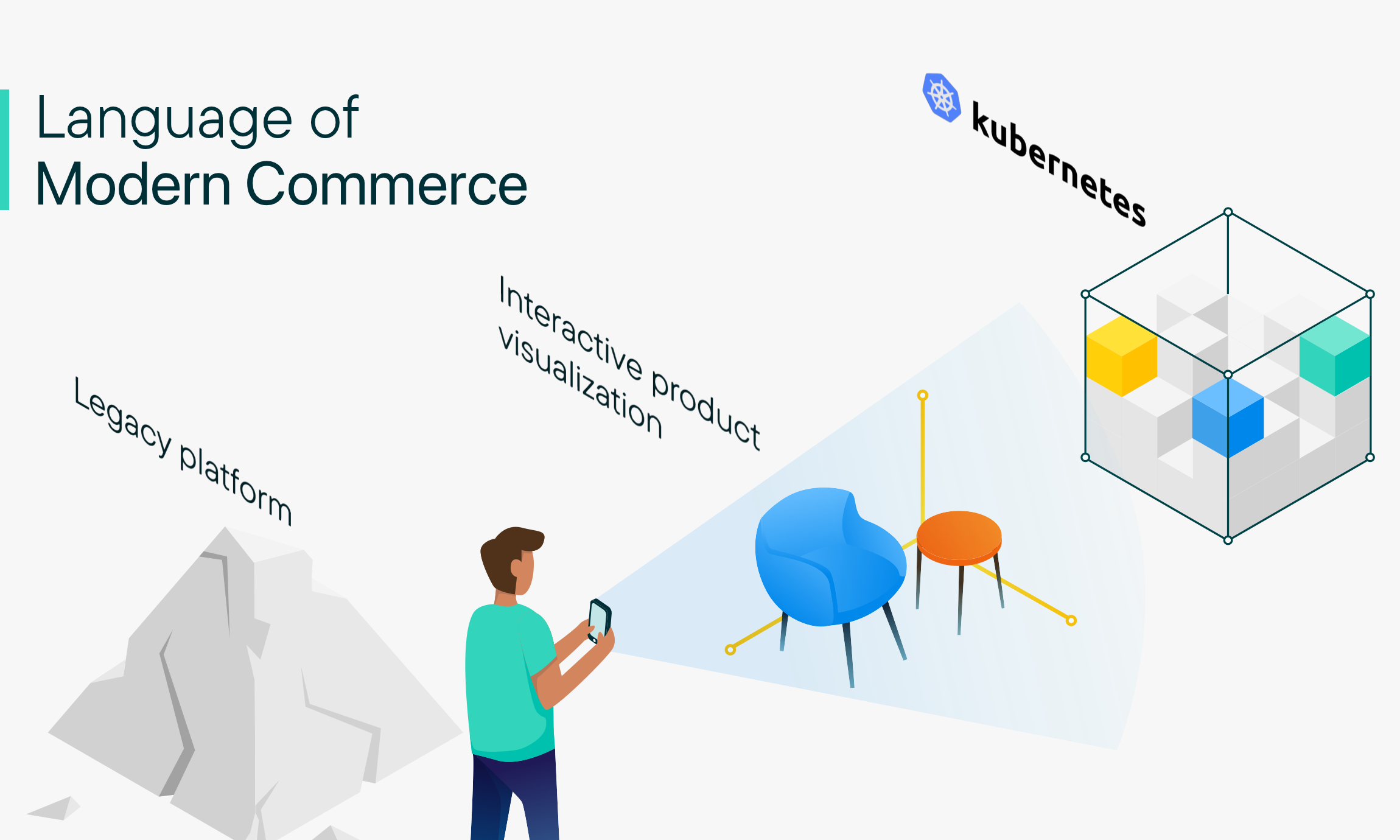This is a detailed colored illustration with the title "Language of Modern Commerce" prominently displayed at the top on a gray background. At the bottom of the image, there are several smaller illustrations. On the left, there is a pyramid-like structure labeled "Legacy Platform" upon a rock. In the center, a man wearing a green shirt and blue pants is depicted holding a cell phone, which shines light onto a blue chair and an orange round table, captioned as "Interactive Product Visualization." To the right, there is a large, semi-transparent square containing three smaller colored squares (yellow, blue, and green) with the text "Kubernetes" above them. Additionally, in the top right-hand corner, there is a logo with the text "Coop Permanence" alongside a blue logo.